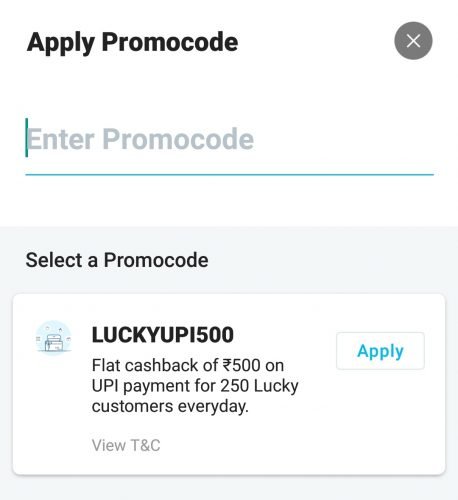The image depicts a promotional pop-up box on a website page. The box features an "X" button in the upper right corner, represented by a circle with an "X" in the center, allowing users to close the pop-up. In the upper left, the text "Apply Promo Code" is prominently displayed. Below this heading, there is a text box containing light gray placeholder text that reads "Enter Promo Code," with a blinking text cursor highlighted in light green, indicating where users can input their code.

Further down, the instructions "Select a Promo Code" are given, accompanied by a smaller pop-up box that contains the code "LUCKYUPi500." Below this code, a message states, "Flat cashback of $500 on payments for 250 lucky customers every day." Adjacent to this, there's a link labeled "View T&C," presumably providing terms and conditions related to the promotion. At the very bottom, aligned to the right, is a clickable "Apply" button. This promotional pop-up is designed to inform users about the opportunity to receive a flat cashback of $500 if they are among the 250 lucky customers each day.